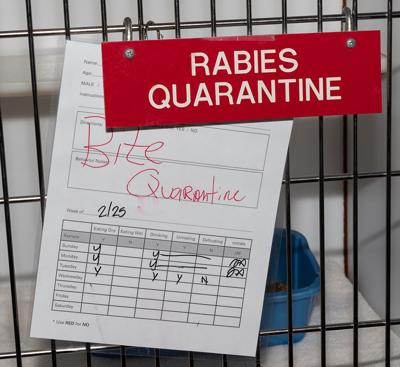This detailed and close-up image shows a small, perfectly squared animal cage with thin black bars. The dominant feature is a red sign with white capital letters stating "Rabies Quarantine," divided over two lines. Behind this sign, a partially obscured piece of paper shows handwritten notes in red ink that read "Bite Quarantine" at the top. Below, a black and white chart is visible, potentially used for tracking details about the animal, such as medications or feeding times, with the handwritten date "2-25" (February 25th). Inside the cage, there's an aquamarine-colored plastic container, which might be a food bowl or litter box, partly obscured by the paper. The floor of the cage appears to have a soft, rug-like material, though the actual animal remains out of sight. The background features a plain white wall, enhancing the focus on the cage and the quarantine signs.